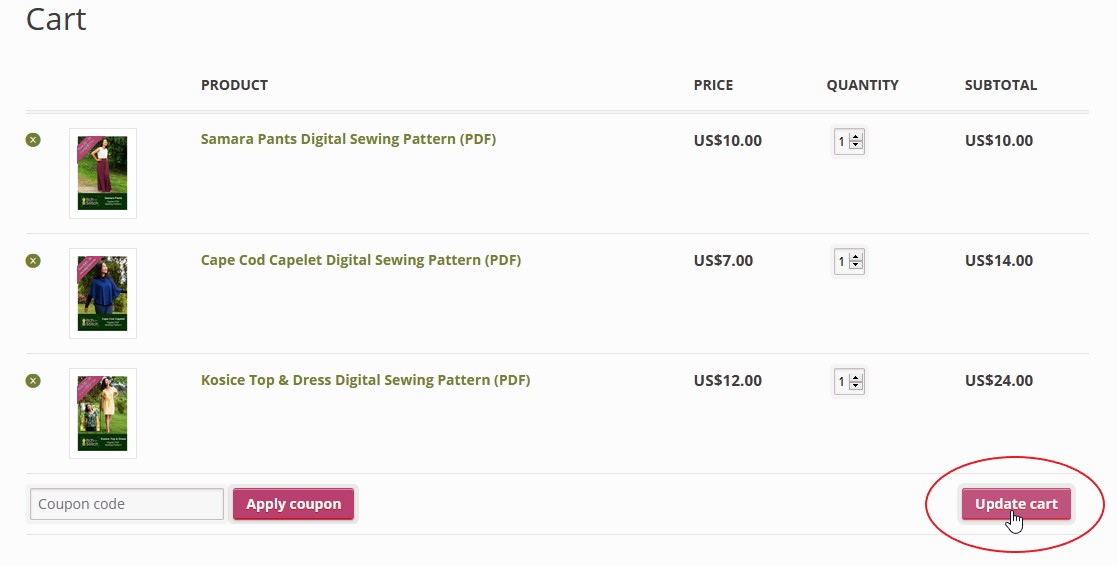This screen capture showcases the cart section of a website's checkout process, highlighting a customer's selection of three different digital sewing pattern PDFs. 

1. **Product Details:**
   - **Item 1:** "Samara Pants Digital Sewing Pattern PDF" priced at $10 with a quantity of one.
   - **Item 2:** "Cape Cod Capelet Digital Sewing Pattern PDF" priced at $7 with a quantity of one.
   - **Item 3:** "Co-Sized Top and Dress Digital Sewing Pattern PDF" priced at $12 with a quantity of one.

2. **Layout:**
   - Each item is aligned in three distinct rows from top to bottom.
   - On the far left of each row, there is an image of the respective product.
   - The product name is displayed in green letters next to the image.
   - The price for each item is listed in clear black lettering.
   - A quantity selection dropdown allows the user to adjust the number of each item they wish to purchase.
   - The subtotal for each product is indicated at the end of the row on the right.

3. **Additional Features:**
   - Directly below the item list, there is a text box for entering a coupon code, which is shown in gray text. Accompanying this text box is a pink "Apply Coupon" button for users to apply any discounts.
   - On the far right, there is an "Update Cart" button that is highlighted with a red circle, providing the option to refresh the cart contents after making changes.

4. **Summary:**
   - The detailed arrangement ensures a clear and transparent shopping experience, enabling the user to easily review their selected items, prices, apply discounts, and update their cart as necessary.